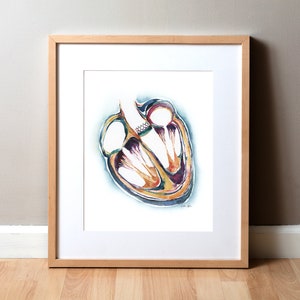The image showcases a framed print resting on a wooden floor with a gray baseboard and wall in the background. The frame is a light wood, almost tan, accentuating the overall aesthetic of the photo. The print itself is highly abstract and vibrant, featuring a white background that highlights the intricate and bold use of yellow, deep purple, orange, and blue hues. The subject of the artwork is open to interpretation: while some perceive it as a dissection of a brain due to its vivid colors and complex shapes, others see mysterious, elongated faces with deep-set eyes. Additionally, there are interpretations suggesting it represents the anatomy of a heart, given its general shape and intricate line work reminiscent of anatomical drawings. Overall, it is a captivating and artsy print, striking a balance between anatomical precision and surreal abstraction.